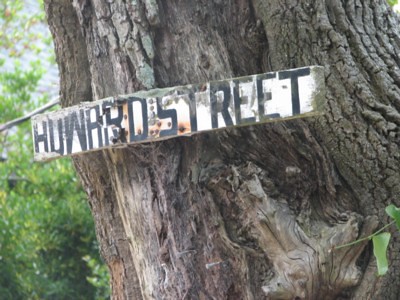The photograph captures a close-up view of a massive, ancient tree trunk. The landscape-oriented image is dominated by the textured bark of the tree, which takes up more than 80% of the frame, stretching diagonally from right to left and extending towards the top of the image. The intricate details of the tree's cracked and weathered bark are clearly visible, showcasing its age and grandeur. Prominently attached to the left side of the trunk is a long, wide, white wooden sign with bold black letters that read "Hewitt Street," indicating its function as a street sign. The background on the left edge of the image reveals a glimpse of green foliage, suggesting the presence of additional trees nearby. The overall composition highlights the majestic presence of the tree while providing contextual clues about its urban environment.